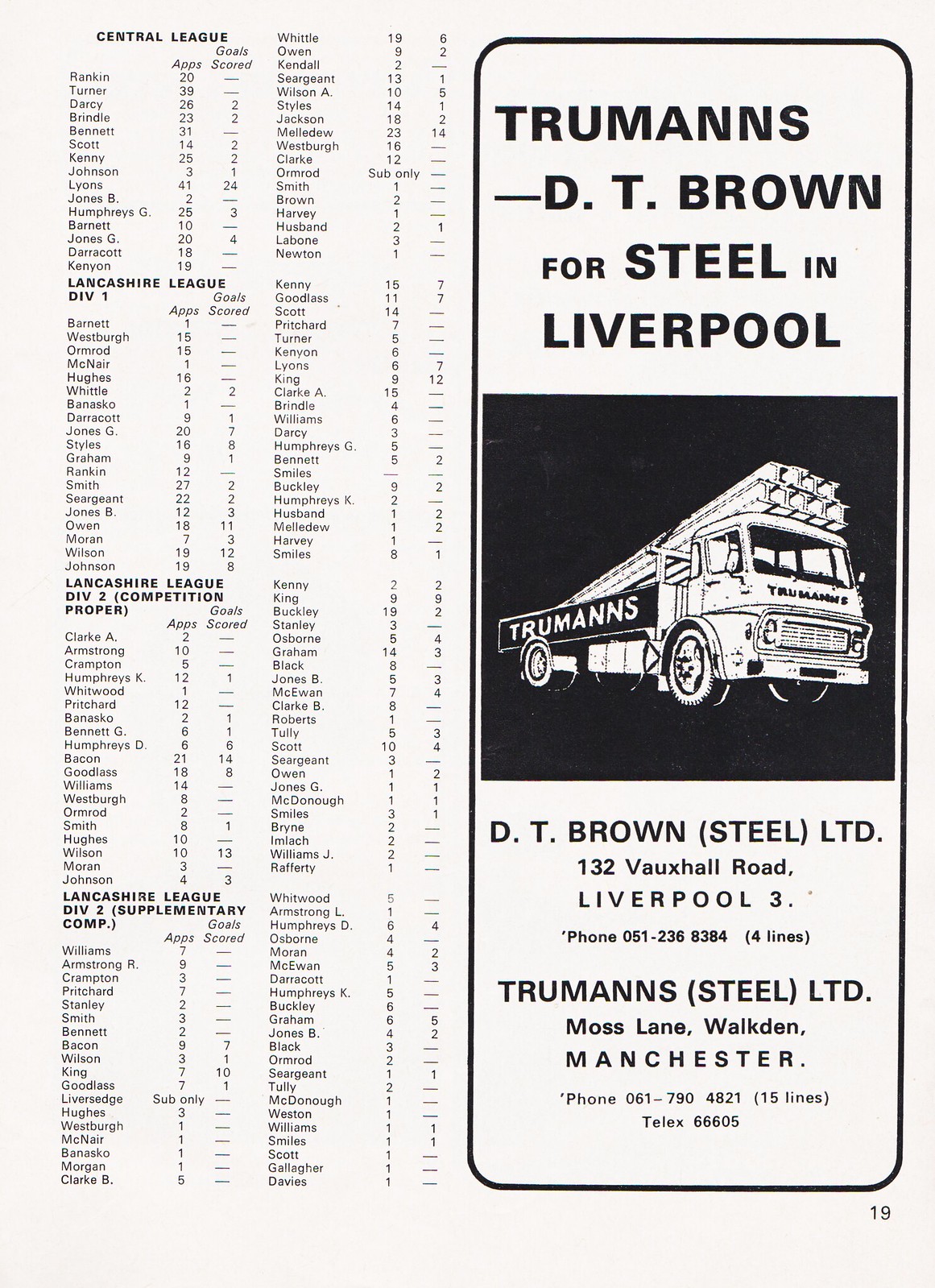The image depicts a vintage newspaper clipping featuring a score sheet for various soccer leagues on the left-hand side and an advertisement on the right. The left-hand side lists player names along with their appearances and goals scored, categorized under different league names including Division 1, Division 2, Division 2 Supplementary, and the Central League. On the right-hand side, there is a large, capitalized advertisement for Truman's D.T. Brown Steel Limited in Liverpool, with additional contact details. The ad includes a black-and-white picture of a truck labeled "Truman's," transporting steel beams. Further details provide the address 132 Vauxhall Road, Liverpool, with a corresponding phone number, as well as information for Truman's Steel Ltd. located at Moss Lane, Walkden, Manchester, accompanied by another phone number.